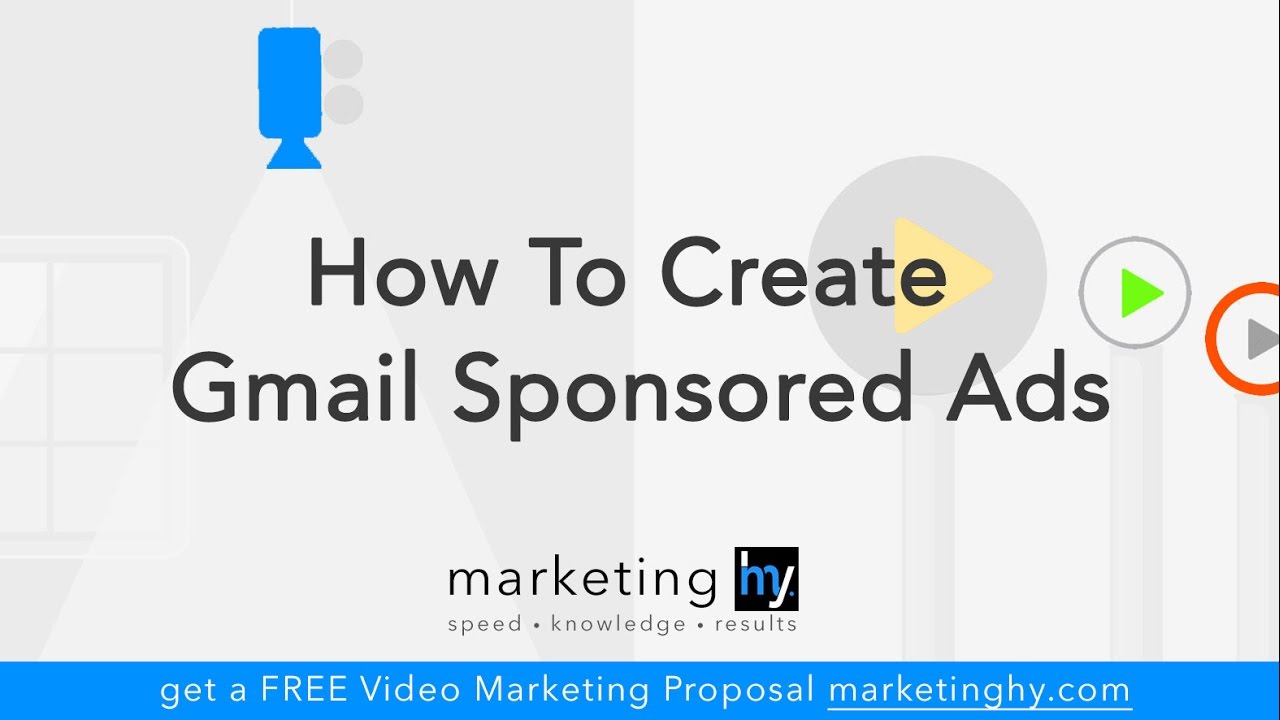The rectangular image, in landscape orientation, features a gradient background shifting from medium gray on the left to a lighter gray on the right. Prominently displayed on the left side is a blue video camera suspended from a white wire at the top center, emitting a burst of light. Adjacent to the camera is a window with layered borders—starting from a medium gray trim, transitioning to a lighter gray, and finally encased in a white border.

To the right, several stick figures resemble the stems of earbuds, each topped with a play button. The first and largest stick figure has a large gray circle and a yellow play button. The second features a gray-outlined circle with a green play button, and the third showcases a thick red circle outline with a gray play button.

In the center, in bold black text, the title reads "How to Create" on one line and "Gmail-Sponsored Ads" on the next. Below this, in a rounded black sans-serif font, appears the word "Marketing."

On the right side of the image, a distinctive black square contains the letters "H" and "Y," with the top of the "H" in white, the bottom in blue, and the "Y" split diagonally—its left side blue and the rest white. Beneath this logo, in rounded gray sans-serif font, are the words "Speed • Knowledge • Results."

At the bottom of the image, a footer with a medium blue background features white text offering a promotion: "GET A FREE" (with "FREE" in capital letters), followed by "video marketing proposal," all underlined with the URL "marketinghy.com."